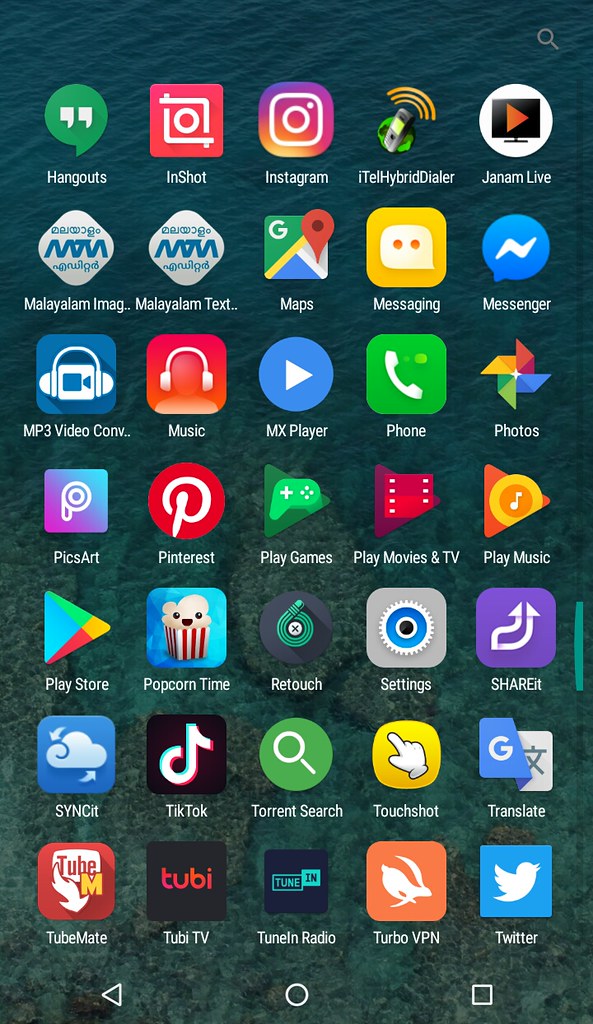A screenshot of a smartphone's home screen, likely an Android device, featuring a captivating ocean-themed wallpaper. The background showcases a dark blue ocean with hints of coral or a shallow seabed visible at the bottom half of the image. The screen is organized into 5 columns and 7 rows of app icons. In the top right corner, a magnifying glass icon indicates a search function. At the bottom, there are three navigation symbols: an arrow for 'back,' a circle for 'home,' and a square for 'recent apps.' A thin, green scroll bar can be seen on the right side, positioned about two-thirds down the screen. App icons are densely packed, with notable ones including Instagram at the top and the classic blue-and-white bird logo for Twitter at the bottom right.